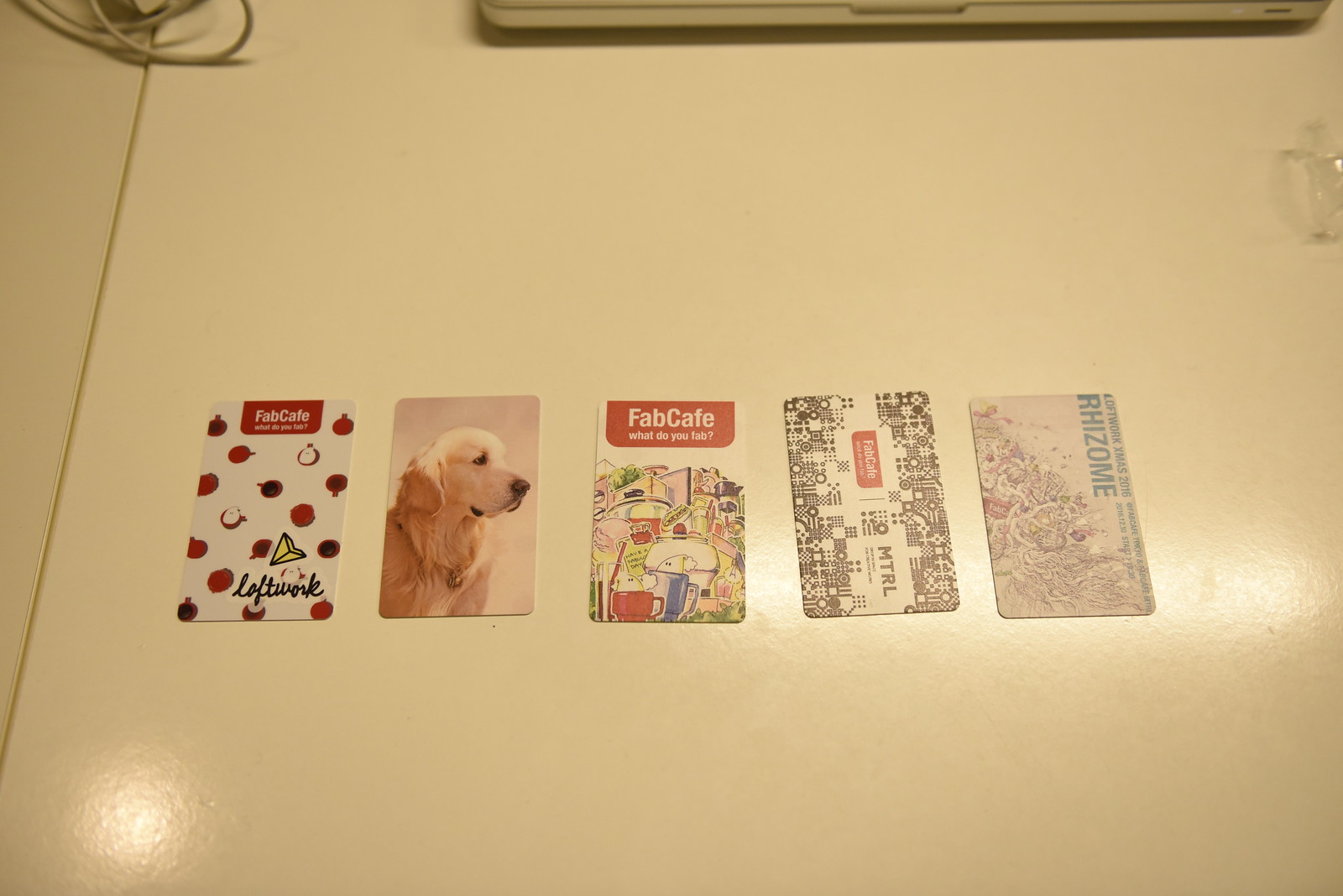This color photograph captures a glossy white table surface reminiscent of high-gloss paint, possibly reflecting light, giving it a scrubable appearance. At the very top edge of the image, there's a slim section of what is likely a laptop, hinting at a digital workspace setting. In the top left corner, part of a small pedestal fan is visible, suggesting a desk environment.

Spread across the table are five rectangular cards roughly the size of a credit card, with rounded corners, akin to the shape of a smartphone screen. The first card on the left features the Fab Café logo in white letters against a red background adorned with apple-like icons and a yellow paper airplane graphic, along with the word "Loftwork". The second card is a color photograph showcasing the right profile of a golden retriever. The third and fourth cards also display the Fab Café logo, with the third featuring various colorful illustrations and the fourth adorned with black and white geometric designs and the term "MTRL". The fifth card, distinctive with its off-white background, blue lettering, and black and white design, prominently displays the word "Rhizome" in all caps.

Overall, this image presents a well-organized and glossy white table or desk with an assortment of visually engaging cards that appear to share themes related to Fab Café and the creative or tech industries, accented by subtle elements of a laptop and a desk fan.